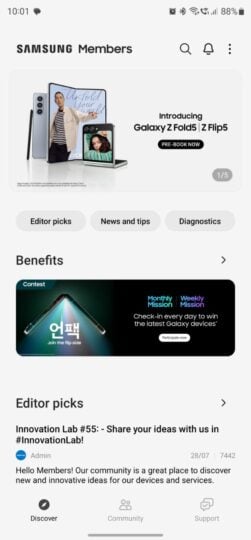This detailed caption describes a screenshot taken from a Samsung Members page. The screenshot is timestamped at 10:01, with the battery level at 80%, Wi-Fi enabled, and Bluetooth disabled. At the top of the screen, next to the timestamp, is a search icon and a notification bell.

The main focus of the screenshot is the announcement and imagery related to the Galaxy Z Fold 5 and Galaxy Z Flip 5, showcasing their unique folding mechanisms, allowing them to be opened and positioned in various ways. Beneath this announcement are several navigational tabs, including "Editor's Picks," "News and Tips," and "Diagnostics."

There's a section labeled "Benefits" with readable and partially unreadable text. Part of it encourages users to check in daily for chances to win the latest Galaxy devices. Below this, the "Editor's Picks" section highlights an initiative called "Innovation Lab #55," inviting members to share their ideas using the hashtag #innovationlab. 

An admin icon follows with the identifier "2807-7442," and welcoming text reads, "Hello member!" It's a message encouraging community participation to discover new and innovative ideas for Samsung devices and services.

At the bottom of the screen are three main tabs: "Discover," "Community," and "Support," with the screenshot indicating the user is currently in the "Community" tab.